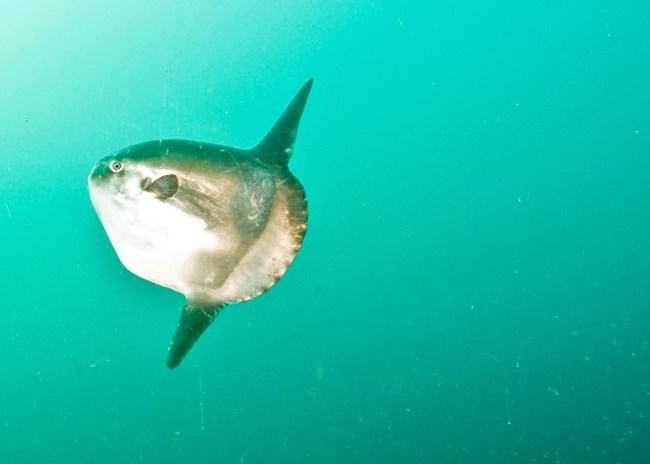The underwater photograph depicts a striking yet elusive scene deep within the ocean's teal and bluish-green depths. Dominating the left side of the frame is a solitary, large sunfish, also known as a mola fish, oriented towards the left. This peculiar fish boasts a roughly bullet-shaped body adorned with small black fins positioned just behind its only visible eye. Notably, the fish lacks a conventional tail, instead featuring two pronounced, pointy triangular fins—one dorsal fin on the top and a matching fin on the bottom—both colored darker than the fish's lighter-hued body. The top of the fish exhibits a strip of darker coloration, while its lower half transitions to a lighter white, particularly towards the back. The water is murky, giving an impression of substantial depth, with no clear light source penetrating through, though there is a subtle flash reflection on the fish, potentially from the photographer's equipment. The backdrop of the image is an enigmatic aqua blue, devoid of any other marine life, enhancing the sense of isolation and introspection of this majestic mola fish, seemingly caught mid-swim, perhaps even startled by the photographer's sudden appearance in its serene underwater world.